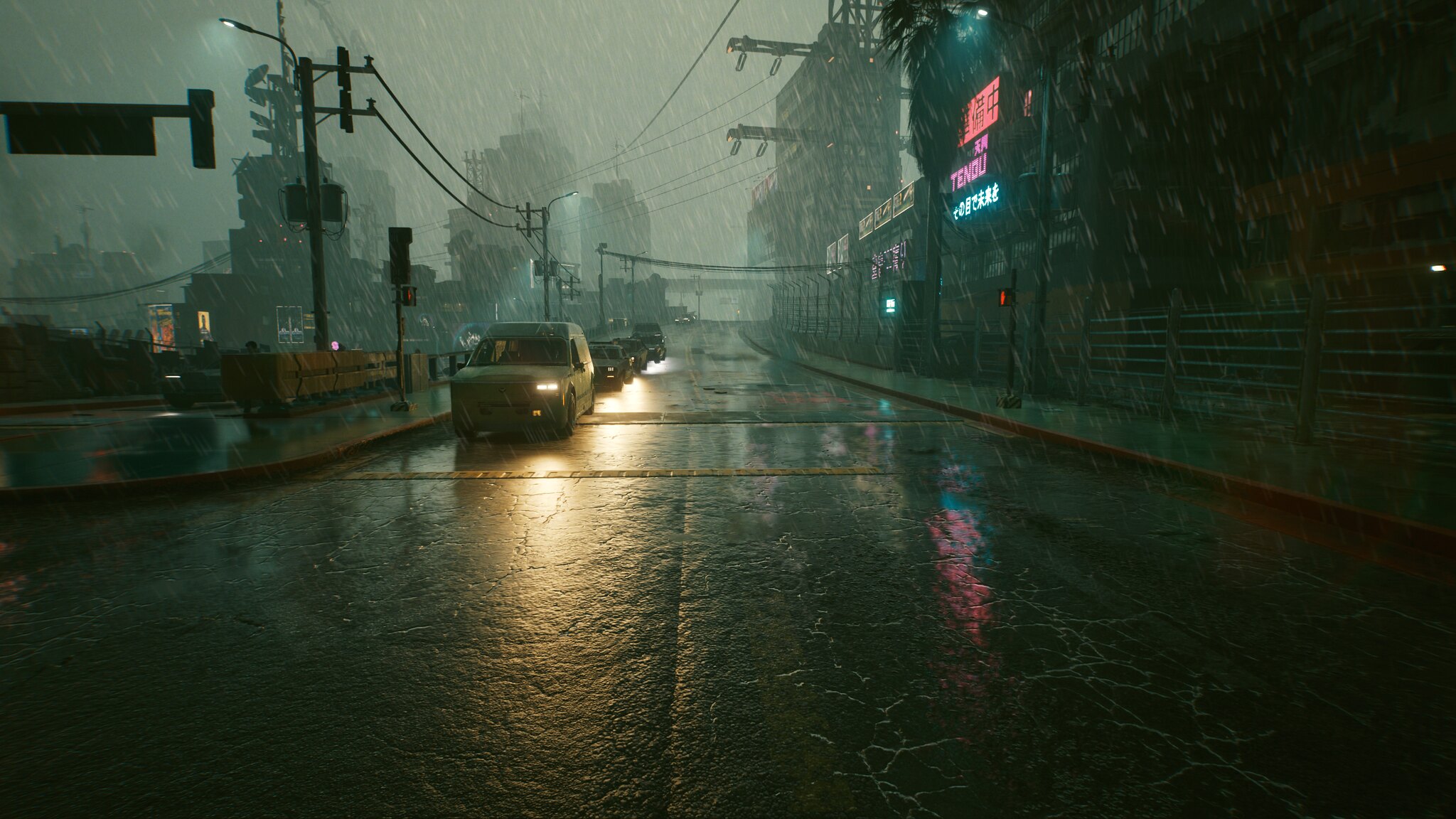A highly detailed, high-definition image reminiscent of a cinematic video game or animated film portrays a stormy, rain-soaked urban street at night. The scene captures a straight road stretching from the foreground into the distance. On the left side, a line of cars, their headlights piercing the gloom, reflects off the glistening wet road, emphasizing the heavy rain. The relentless downpour creates a pervasive dark, gray atmosphere, enhancing the moodiness of the scene. To the right, a series of neon signs glow vibrantly from storefronts, offering a stark contrast to the otherwise somber environment. Various cables and telephone lines crisscross above the street, adding to the urban complexity and deepening the sense of immersion in this stormy, nighttime setting.